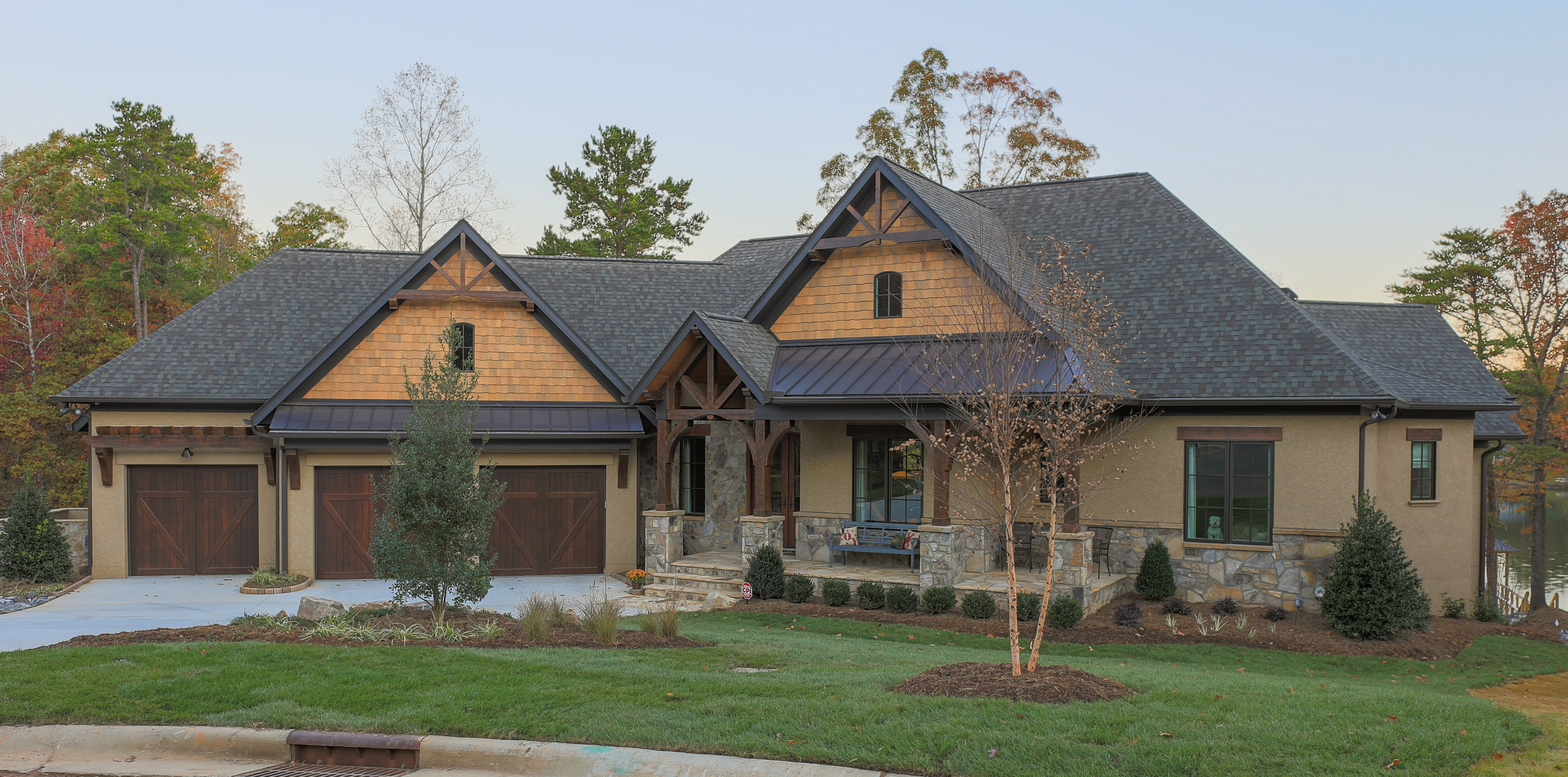The image portrays a charming, suburban house with a Western-style and farm aesthetic, set against a backdrop of an autumn landscape with changing leaves and a setting sun. The house features multiple architectural elements including a dark gray, asphalt-shingled roof with two pitches—one extending over the main house and another over the attached, multi-door garage. The garage doors are distinctive, dark-stained wooden farm doors, two on the main garage and two additional doors to its left.

The exterior walls are a tan or muted brown color, accented by a stone veneer base in shades of gray and beige. Deep-stained wooden beams and posts support the porch, which features stone steps and stone-pillared columns. The porch area is furnished with a blue bench adorned with pillows, as well as a couple of black chairs, creating a welcoming outdoor space. Trees and shrubs are thoughtfully planted around the house, with a green grass lawn extending out to a nearby lake or pond seen on the right side. The sky is clear blue, capturing the warm glow of the sunset, further enhancing the picturesque setting of this beautiful, sizeable residence.